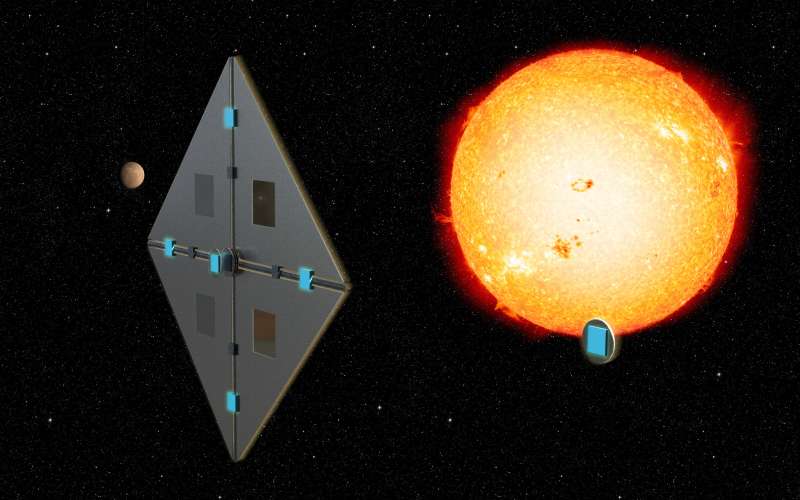The image depicts a vivid space scene featuring a prominent orange-colored celestial body, distinctly identified as the sun. The sun emits a radiant reddish-orange glow with flares extending from its outer regions, and its core shines brightly with a mix of white, yellow, and orange hues. Positioned to the left of the sun is a large, diamond-shaped silver panel divided into four triangular sections, each adorned with bright neon blue brackets and containing small rectangular boxes. This panel, resembling a solar reflector, appears designed to harness the sun's energy. To the left of this panel is a significantly smaller spherical planet, possibly Mercury or Venus. The scene is set against a backdrop of a black space littered with white speckled stars, enhancing the contrast and dramatic effect of the glowing sun and reflective panel. The overall image exudes an otherworldly and dynamic feeling, hinting at a possible depiction of space exploration or energy harvesting technology.